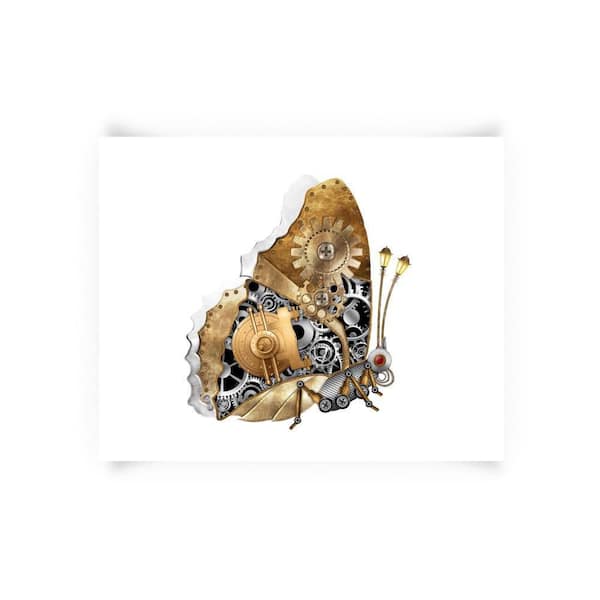This detailed steampunk-inspired artwork showcases a mechanical butterfly with intricately crafted features. The butterfly's wings are made out of metal, composed of an assortment of gears and cogs, epitomizing the essence of steampunk design. Its robust body is constructed from steel, with the delicate legs fashioned from bronze, enhancing the metallic charm. The antennas are ingeniously designed as street post lamps, one slightly bent forward, adding a whimsical touch. The butterfly's head is dominated by a large, red robotic eye, and it has a spiral proboscis suggestive of a spring, giving it a playful and almost lifelike quality. The creature's joints are depicted as small wheels and screws, emphasizing its mechanical nature. Set against a plain white backdrop, the image highlights the striking combination of brass, gold, and silver hues, reminiscent of the intricate style of Gustav Klimt.